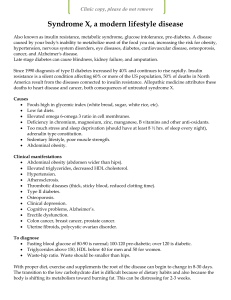This low-resolution screenshot depicts a document, potentially from a peer-reviewed study, which is challenging to read due to its poor quality. At the top of the document, a banner is visible, possibly stating "Clinic Copy - Please Do Not Share or Distribute." The document's title, bolded in black font, reads "Syndrome X: A Modern Lifestyle Disease." The body of the text comprises one to three paragraphs discussing Syndrome X. A bulleted list is embedded between the second and third paragraphs, likely detailing headings such as "Causes," "Clinical Symptoms," and "Diagnosis." The article appears to explore the origins, clinical manifestations, and diagnostic criteria of Syndrome X, aiming to provide insights into its causes and potential treatments.